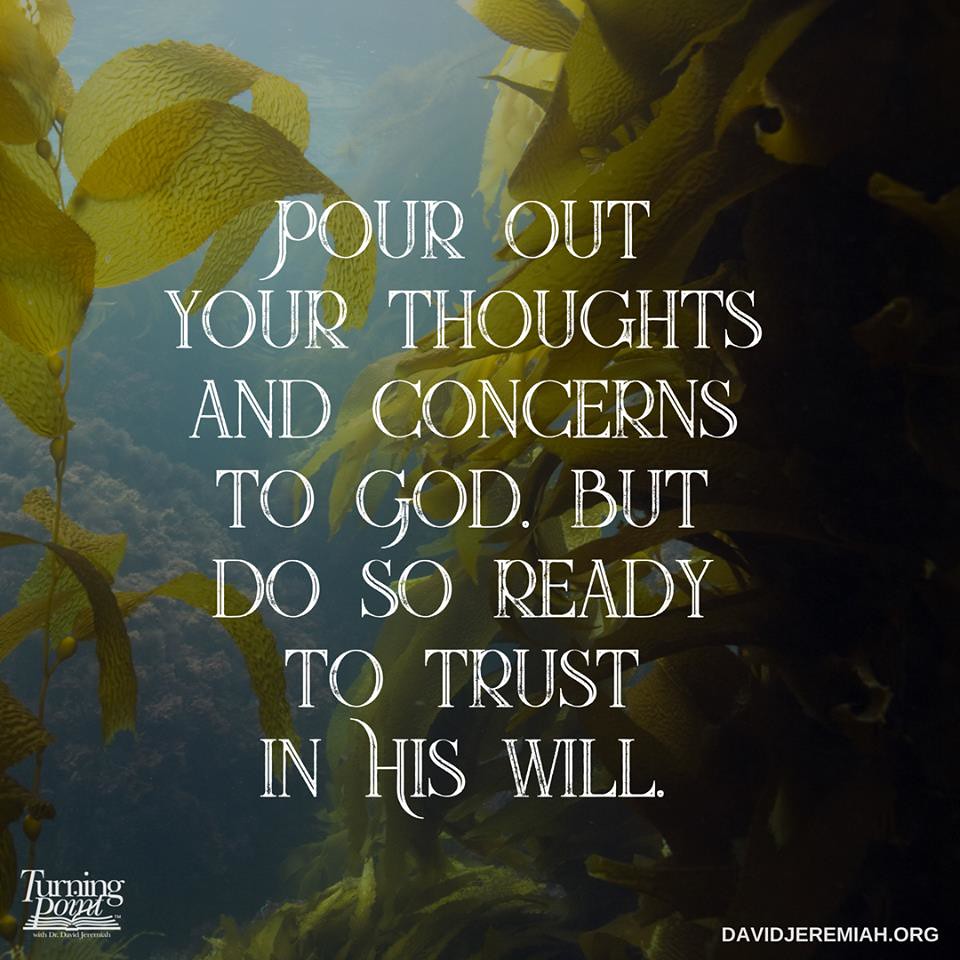The large square image features an underwater scene, giving the impression of being taken by a scuba diver amidst a coral reef. The background is a mix of dark blue and grayish-blue hues, suggestive of clear but slightly murky water. On the left side, there are large, out-of-focus green leaves, extending from the upper left corner down the side. The right half of the image shows a dense area of underwater vegetation or seaweed, creating a rich, natural texture.

Prominently displayed in the center of the image in all caps, white text, is the inspirational message: "POUR OUT YOUR THOUGHTS AND CONCERNS TO GOD, BUT DO SO READY TO TRUST IN HIS WILL." In the lower left corner, there is a logo featuring the name "Turning Point" alongside an open book icon, both in white text. The lower right corner contains the URL "DAVIDJEREMIAH.ORG," also in white, identifying the associated ministry.